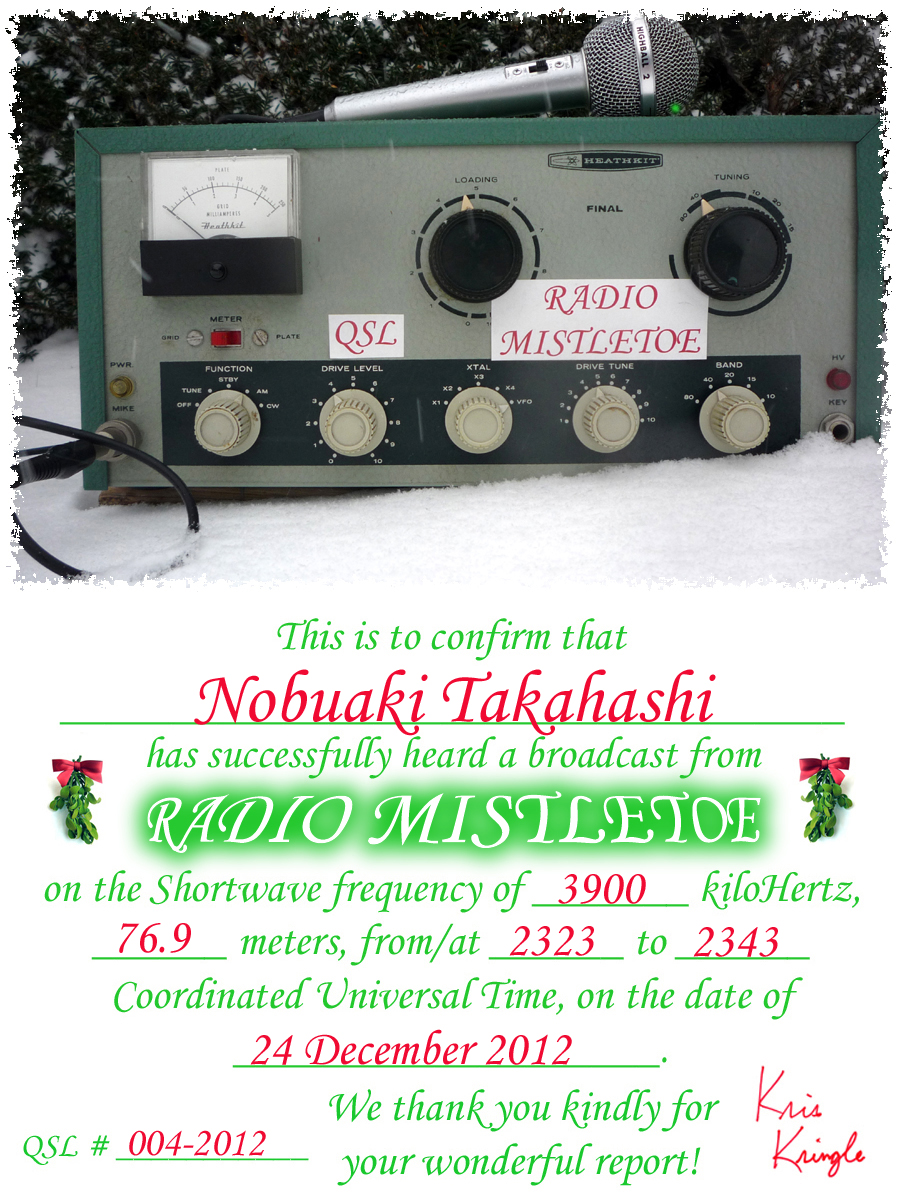This image consists of two main sections: a photograph on the top and text below it. The top features an old-time radio with a microphone, characterized by its beige and black knobs, including five buttons and two larger dials, as well as a sound frequency bar on the left beneath the microphone. The radio is adorned with stickers bearing red letters on a white background; one reads "QSL" and another "Radio Mistletoe." This setup sits on snow, with snow-dusted greenery visible in the background.

Below the radio, green and red text provides a detailed confirmation: "This is to confirm that Nabuaki Takahashi has successfully heard a broadcast from Radio Mistletoe on the shortwave frequency of 3,900 kilohertz (76.9 meters) from 2323 to 2343 Coordinated Universal Time on December 24, 2012." There are two images of mistletoe flanking the "Radio Mistletoe" text. Additional details about the broadcast, filled in with red handwriting, include QSL number 004-2012. The confirmation is signed by Chris Kringle, enhancing the festive atmosphere of this Christmas-themed broadcast advertisement.